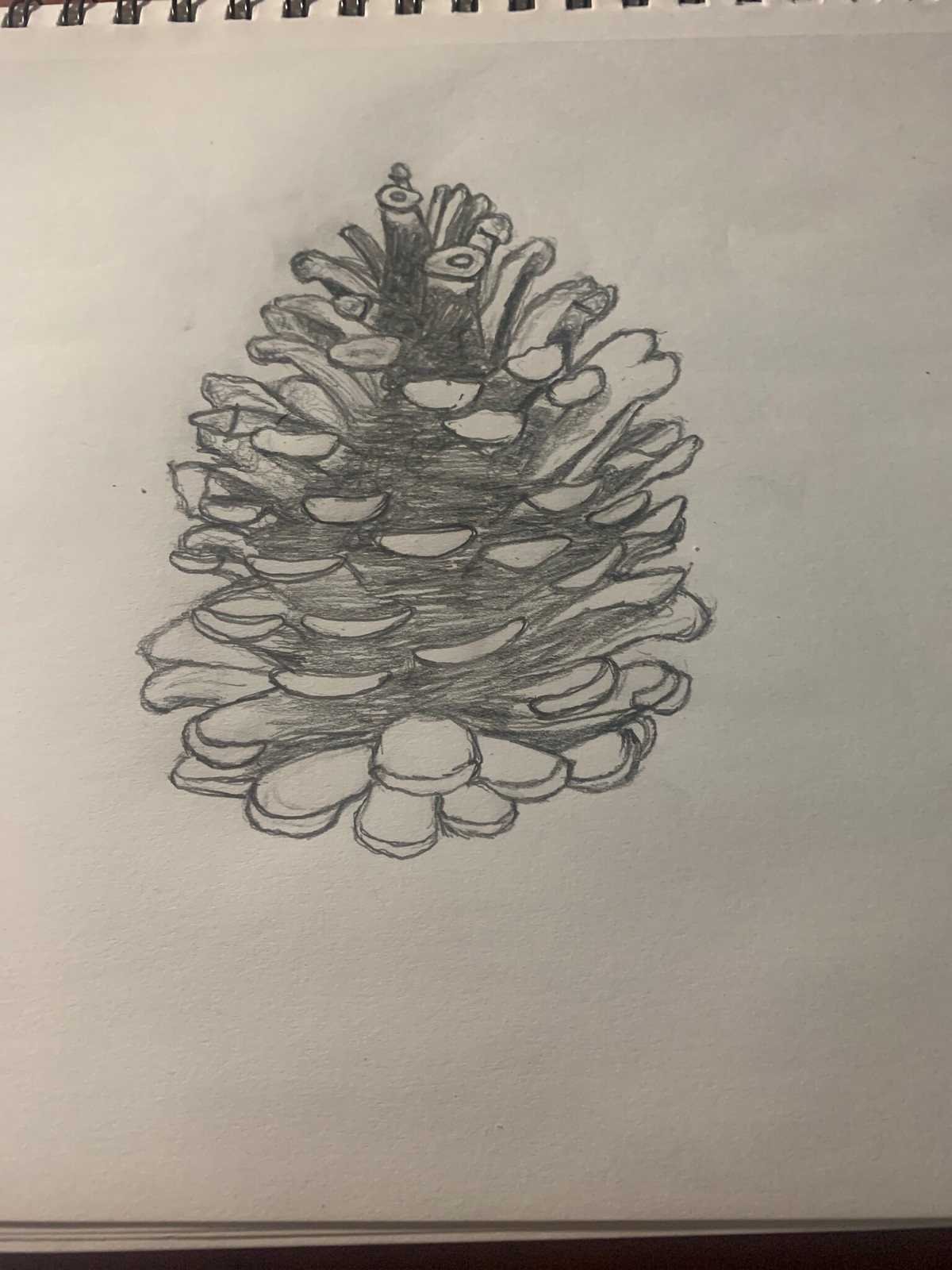The photograph showcases a meticulously hand-drawn pine cone, rendered on a pristine piece of white paper using pencil. This dry pine cone illustration features relaxed and open scales, with the artist employing intricate shading techniques to create depth and texture. The interior of the pine cone is densely shaded, offering a stark contrast to the lighter, almost white tips of the scales, emphasizing the natural gradient and form. At the top of the pine cone, multiple stem-like structures extend outward, adding to the overall realism and detail of the artwork.